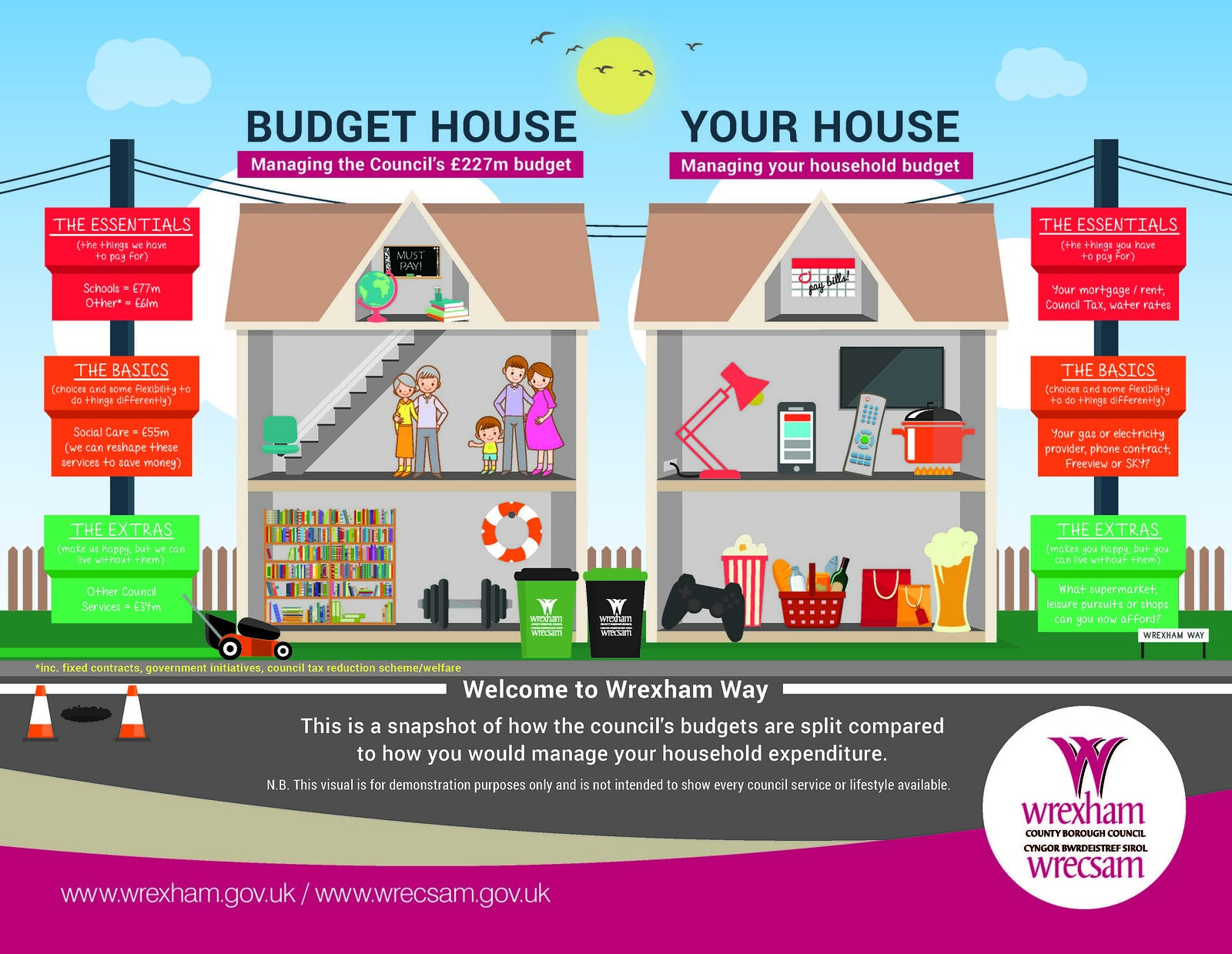This detailed, colorful infographic titled "Welcome to Wrexham Way" serves as a visual comparison between managing the Council's £227 million budget and a typical household budget. 

The upper portion of the image features a blue sky with two clouds, a yellow sun, and birds flying in a V shape. Below this, the infographic depicts two houses side by side. The left house, labeled "Budget House," represents managing the Council's budget and includes various items such as a family, a stairlift, a bookshelf, weights, a life preserver, and two waste cans placed out front. 

The right house, labeled "Your House," symbolizes managing your household budget and features items like a calendar, a pot on a flame, a remote control, a cell phone, a desk lamp, a video game controller, popcorn, shampoo, gift bags, and a drink. 

This snapshot compares the essentials, basics, and extras found in both budget types, visually demonstrating how council budgets are allocated compared to household expenditures. Please note that this infographic is for demonstration purposes only and does not include every Council service or lifestyle option.

The bottom right corner features an advertisement for the Wrexham County Borough Council, with the official website, www.wrexham.gov.uk, listed at the bottom left.